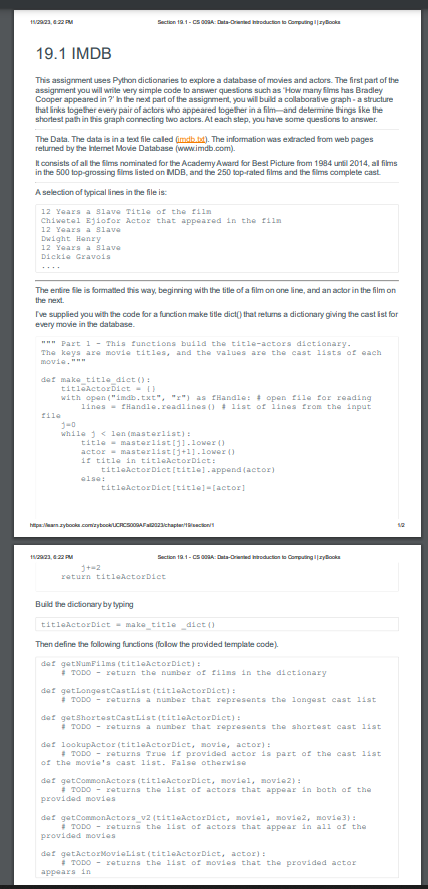This is a computer printout displayed on a white background, primarily featuring black text. The text at the top reads "19.1 IMDB" and specifies the parties involved in an agreement concerning the database of movies and actions. The document elaborate on the specifics of these movies and their respective actions, including detailed explanations. One segment of the text stands out in orange and is underlined, likely to highlight its importance.

The printout references the movie "12 Years a Slave," classifying it under specific criteria that need to be addressed. There are directives relating to the structure and order of the information, but the font size is quite small and requires enlargement for better readability. As noted, the document includes a supplied code for some function, which extends into subsequent sections of the printout. Part two appears to consist mainly of printed computer information, and part three continues in the same vein, requesting additional computer-related details.